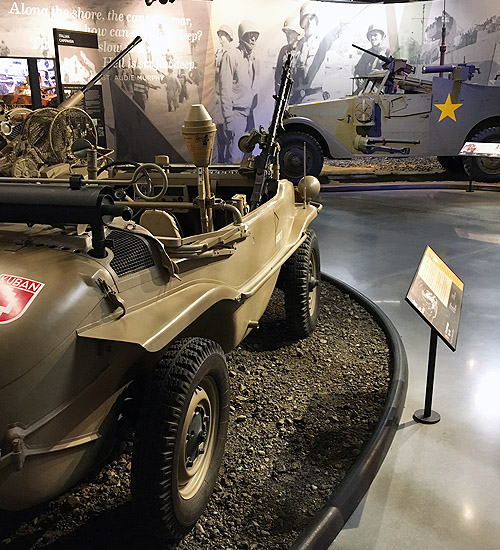In this indoor image, taken at a military museum, there is a prominent display featuring a vintage military vehicle. The central vehicle appears to be a tan-colored convertible Jeep with black tires, situated on a dirt-covered surface surrounded by a berm. This Jeep, reminiscent of military transport, lacks a roof and holds significant historical importance. In the background, the wall is adorned with a graphic mural of military personnel dressed in uniforms and helmets, enhancing the historical and immersive atmosphere of the exhibit. Additionally, another gray Jeep, marked with a yellow star, stands in front of the mural. Above this scene, signage reads "Along the Shore," contributing to the thematic setting of the display.